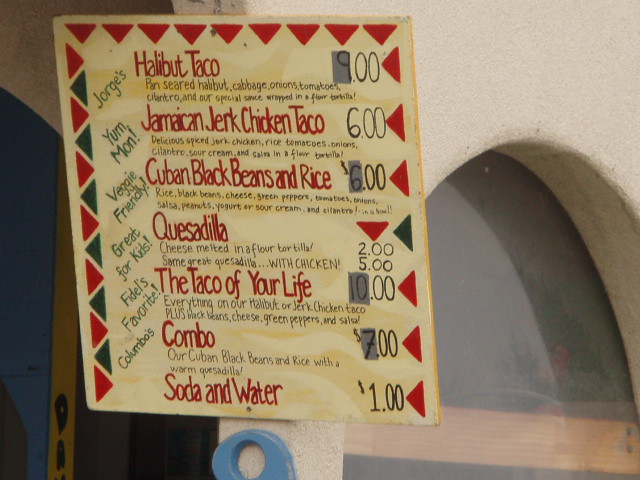The image features a menu posted on the side of a building constructed from concrete blocks and fashioned into a charming arch, which also houses a visible window. The menu is displayed on a vibrant yellow card, embellished with festive green and red triangles. The tantalizing offerings include a Halibut Taco priced at $9, a Jamaican Jerk Chicken Taco for $6, and a Cuban Black Beans and Rice dish also for $6. A Quesadilla is available in two options: a plain version for $2 and a Chicken Quesadilla for $5. The intriguing "Taco of Your Life" is listed at $10. A combo meal, featuring Cuban Black Beans and Rice paired with a warm Quesadilla, is priced at $7. Additionally, refreshing beverages such as soda and water are each priced at $1.

Down one side of the menu, playful markers in green lettering accompany each item: "George's" for the Halibut Taco, "Yum Mon" for the Jamaican Jerk Chicken Taco, "Veggie Friendly" for the Cuban Black Beans and Rice, "Great for Kids" for the plain Quesadilla, "Fidel's Favourite" for the Chicken Quesadilla, and "Columbo's" for the combo meal, adding a personal and whimsical touch to the descriptions.